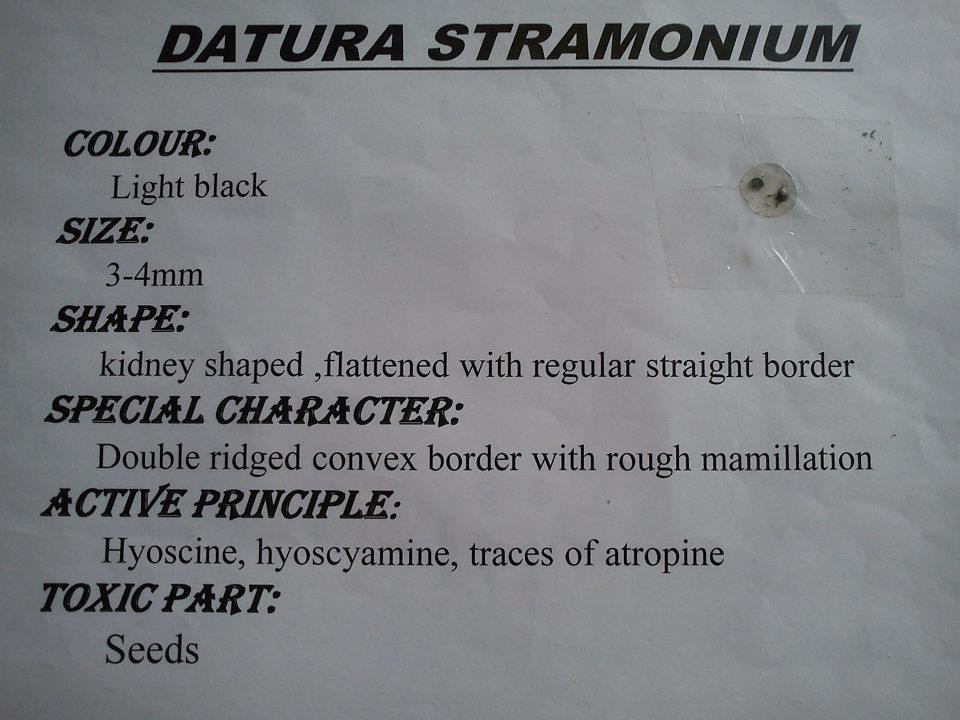The image depicts a printed and slightly crinkled piece of paper with "Datura stramonium" prominently displayed at the top in bold, italicized lettering. The paper appears to have originated from a European country, indicated by the British spelling "colour." Taped on the right side of the paper is a small cluster of seeds. Detailed information about these seeds is listed on the left side of the paper, starting with their description: color – light black, size – 3 to 4 millimeters, shape – kidney-shaped, flattened with a regular straight border. Under the special characters section, it mentions a double-ridged convex border with rough mammalation. Further down, the active principle section lists hyosin, hyosciamine, and traces of atropine, indicating the toxic nature of Datura stramonium seeds. The overall format is structured with bold headings followed by descriptive text, providing a comprehensive rundown of the plant’s key characteristics and toxic properties.